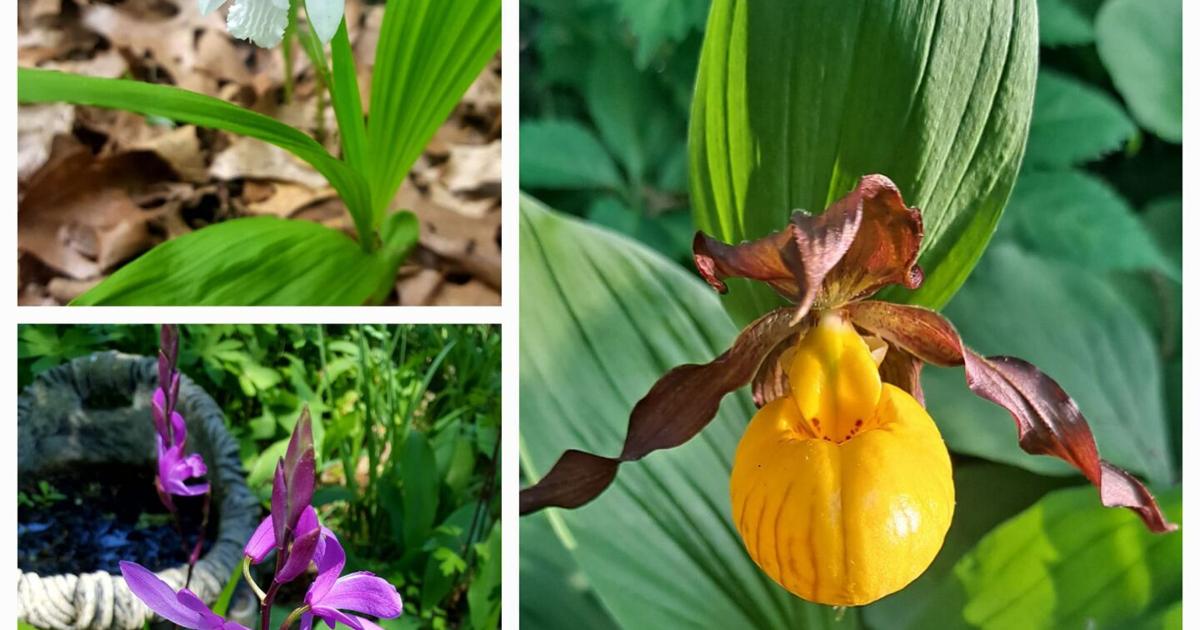The image is divided into three sections: two smaller, side-by-side images on the left, and a larger, single image on the right. At the top left, there is a close-up of green shoots emerging from a ground covered in brown, dried leaves. The lower left image features vibrant greenery with two prominent purple flowers, one in the center and a smaller one to the right, backlit by sunlight adding a shine to the foliage. This section also includes details of a gray, bowl-like structure, possibly a fountain, in the background. The larger right-side image showcases a striking yellow flower with a bulbous, almost squash-like base and brownish-red leaves extending from it, creating an appearance akin to wings. The background consists of green leaves illuminated by light coming from the right side, enhancing the highlights on both the yellow orb and the brown leaves.